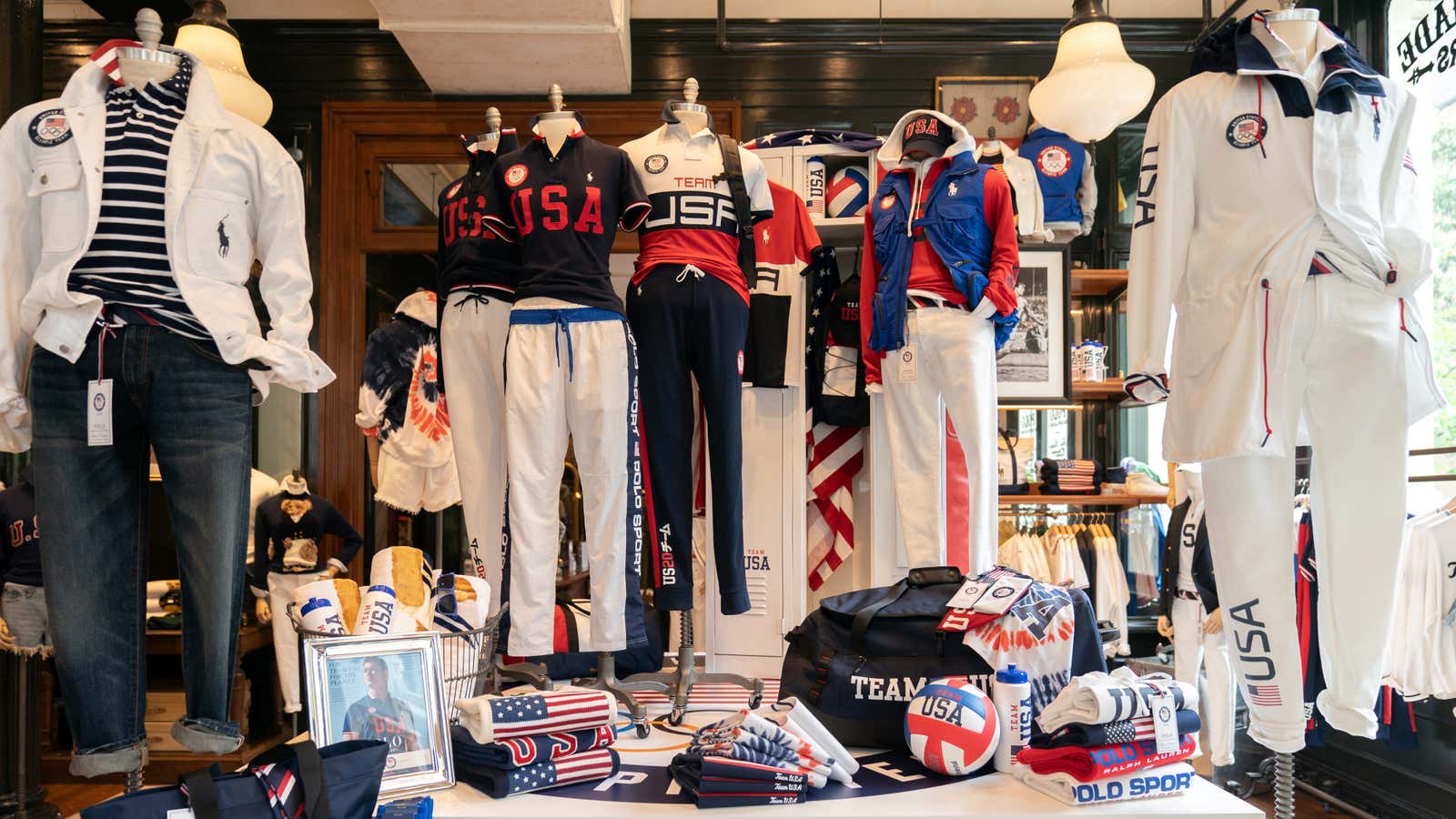The image captures the interior of a store, specifically a boutique or gift shop, with a focus on Olympic-themed items. Dominating the scene is a central display table laden with Ralph Lauren-branded duffel bags, volleyballs with blue, red, and white stripes, towels, and water bottles, all themed around the Olympics. Surrounding the table are headless mannequins dressed in what appears to be official Olympic uniforms, featuring white and navy blue tops with "USA" and "Team USA" emblazoned in red or blue. One standout mannequin is adorned with jeans, a white jacket with horizontal navy blue and white stripes, and a price tag hanging from it. Behind the table, the rear wall is painted black and includes a wooden-framed door, adding contrast to the vibrant merchandise. To the left of the display, a framed portrait of a young man in his 20s, possibly an athlete, wearing a blue "USA" t-shirt is positioned next to a basket filled with additional products. A window on the top right offers a glimpse of greenery outside, further enhancing the store's inviting atmosphere.